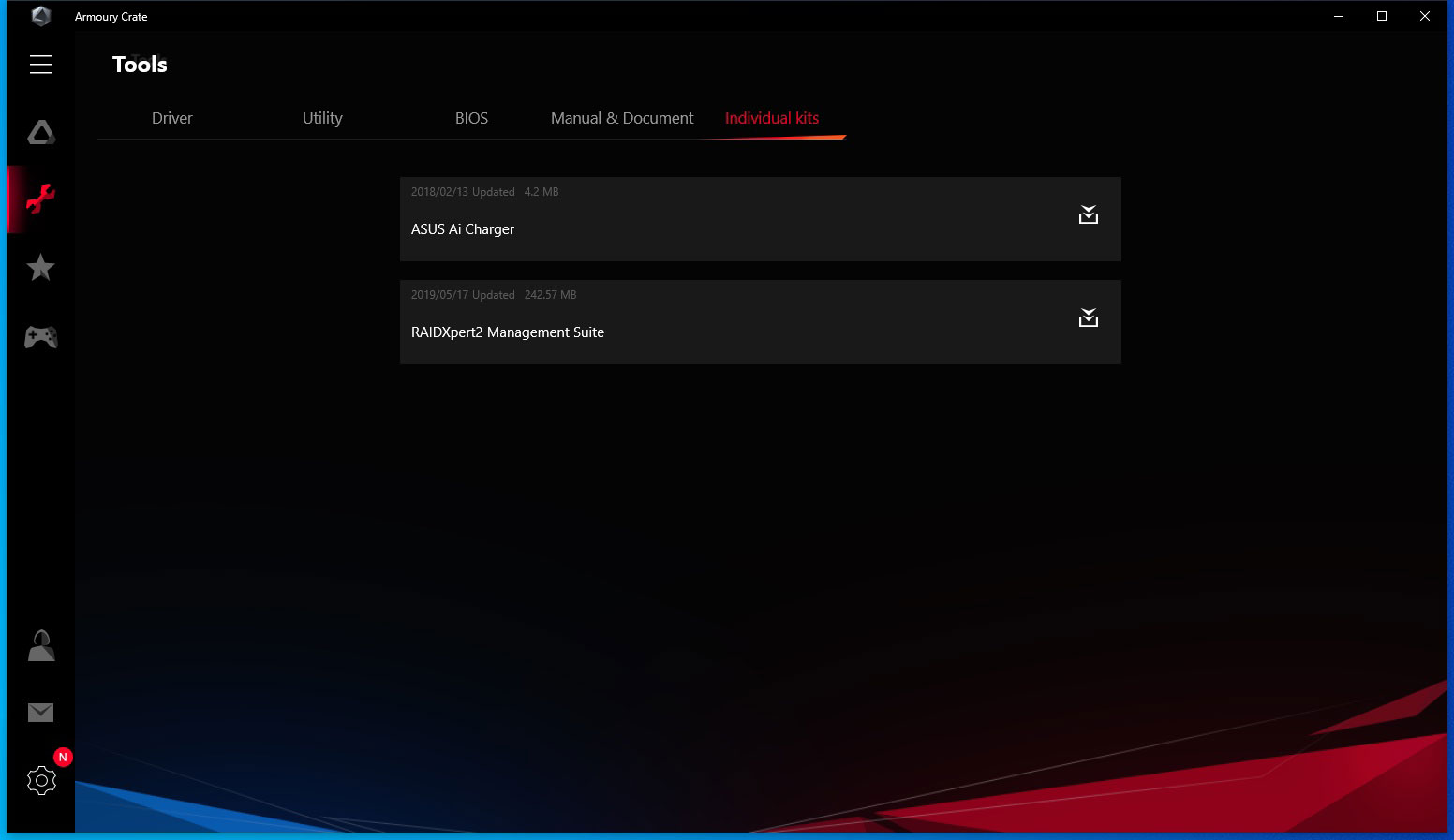Screenshot of a website interface, possibly the Armory Crate application from ASUS. The interface has two menu bars: one on the left and one at the top of the screen. 

The left menu bar features several icons in descending order: a menu button at the top, followed by a triangle, a wrench, a star, a gaming icon, a controller, a gap, a shopping bag, and an envelope icon, with a gear icon for settings at the very bottom. 

The main section of the screenshot is titled "Tools," displaying several categories such as Driver, Utility, BIOS, Manual and Document, and Individual Kits. The focus is on the "Individual Kits" section, highlighting a search for an "Asus AI Charger." Additionally, a "Raid Expert 2 Management Suite" is mentioned below this. It is not clear whether these tools are pre-installed on the device or available for download.